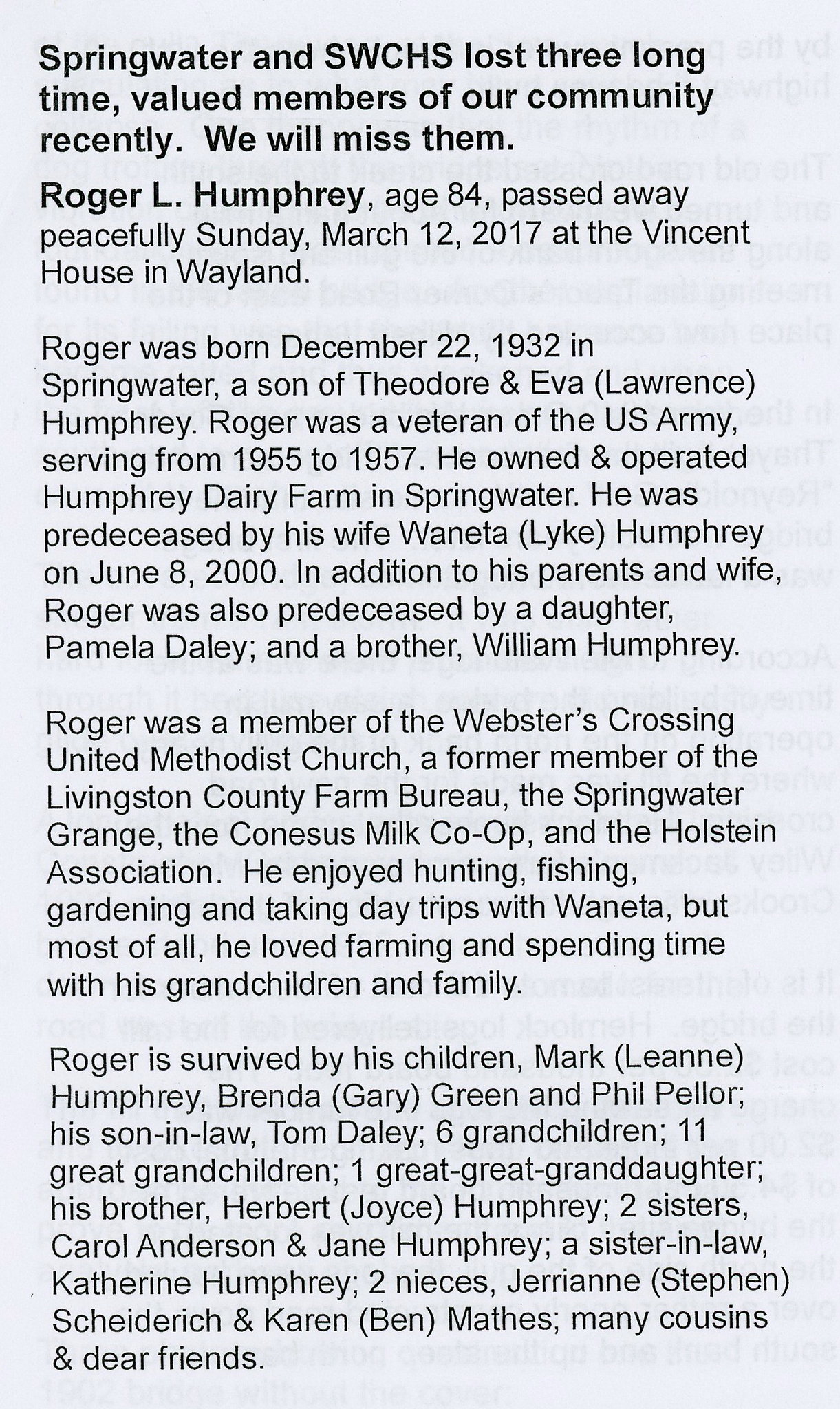The image displays an article titled "Springwater and SWCHS lost three long-time valued members of our community recently. We will miss them." It details the life of Roger L. Humphrey, age 84, who passed away peacefully on Sunday, March 12, 2017, at Vincent House in Wayland. Born on December 22, 1932, in Springwater to Theodore and Eva Lawrence Humphrey, Roger was a U.S. Army veteran who served from 1955 to 1957. He owned and operated Humphrey Dairy Farm in Springwater. He was predeceased by his wife, Juanita Lyke Humphrey, on June 8, 2000, along with his daughter, Pamela Daly, and his brother, William Humphrey. Roger was an active community member, involved with the Webster's Crossing United Methodist Church, Livingston County Farm Bureau, Springwater Grange, Knesset's Milk Co-op, and the Holstein Association. He enjoyed hunting, fishing, gardening, and day trips with his wife, but his greatest love was farming and spending time with his family. He is survived by his children, Mark Leanne Humphrey, Brenda Gary Green, and Phil Peller; his son-in-law, Tom Daly; six grandchildren; 11 great-grandchildren; one great-great-granddaughter; his brother, Herbert Joyce Humphrey; and two sisters, Carol Anderson and Jane Humphrey, along with his sister-in-law, Katherine Humphrey; two nieces, Gerianne Stephen Scheiderich and Karen Ben Mathis; many cousins; and dear friends. The background shows the text through the white paper, though it is not readable.